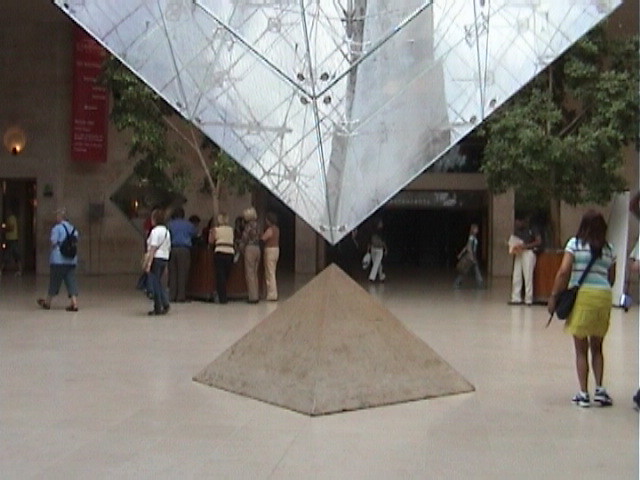In the blurry and pixelated image of the mall concourse, there stands a small, beige pyramid in the center. Balancing just above it, without touching, is an upside-down white triangular prism, creating a striking visual element. Around the pyramid, various people stroll about, contributing to the busy atmosphere of the scene. On the right side of the pyramid, a woman wearing a yellow skirt and a blue and white striped shirt stands near a tall indoor potted tree. To the left, a group of seven individuals forms a circle around another potted tree. Nearby, there is a darkened store entrance, possibly indicating that it is closed. The scene is reminiscent of the entranceway of the Louvre museum in France, complete with help desks and archway entrances to the main parts of the museum, enhancing the overall ambiance of this bustling, indoor space.